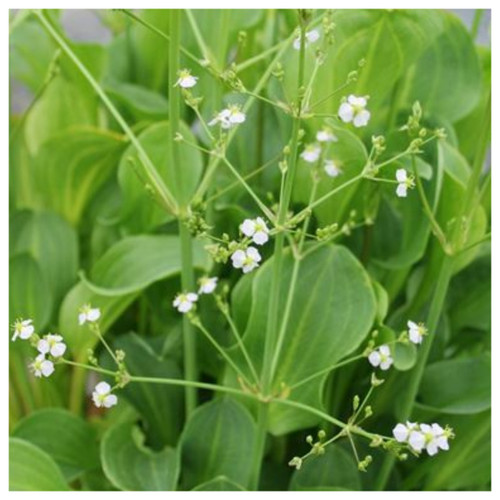The photograph captures a lush garden scene dominated by healthy, large green leaves with pronounced vertical veins, suggesting a well-moisturized and thriving environment. These leaves crowd together, creating a dense backdrop. In the foreground, delicate green stems hold clusters of dainty white flowers. Each flower has three petite white petals surrounding a yellow center with tiny yellow stamens. While some blooms are fully open, others remain as small, green buds, yet to blossom. The flowers are scattered across the image, with noticeable clusters on the bottom left, bottom right, and the top center, enhancing the overall picturesque beauty and hinting at the early stirrings of spring.